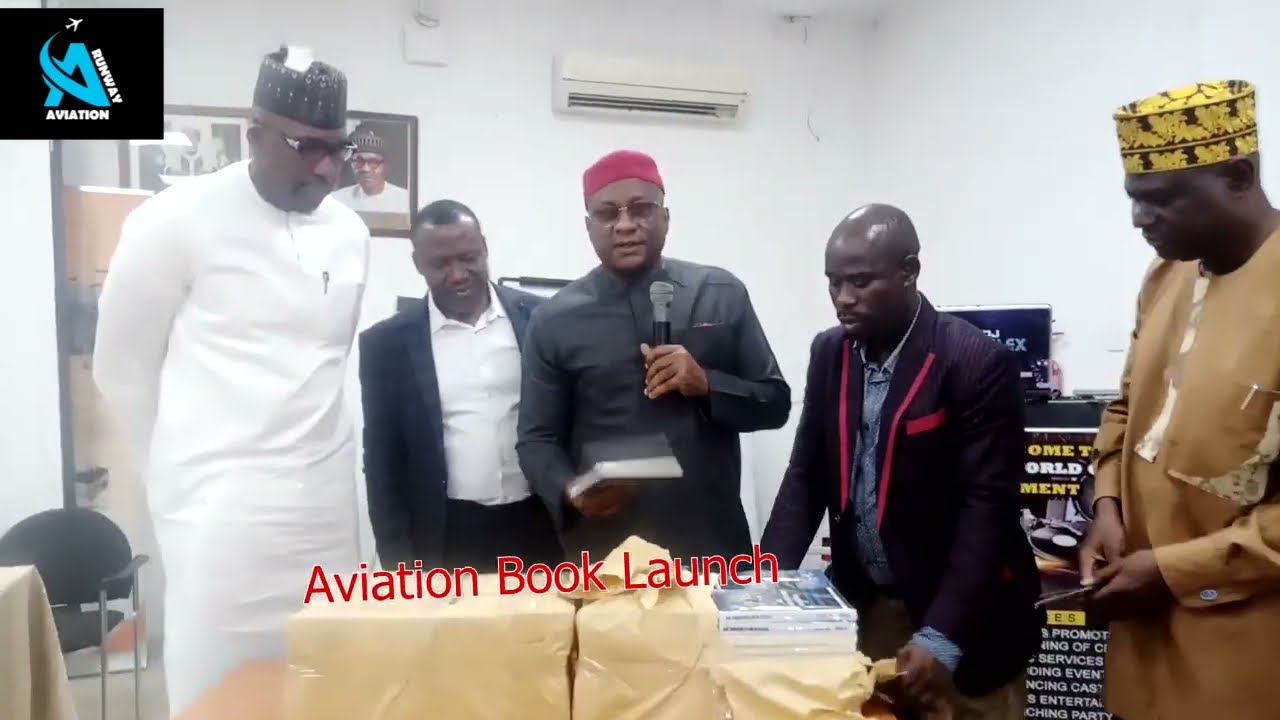The image captures a significant moment at an Aviation Book Launch event titled "Runway Aviation," as indicated by the large text and the airplane graphic making an 'A' at the top left. The event features a group of five African men, each playing a distinct role. On the far left, a tall man wearing glasses and a traditional white African attire with a patterned black round hat stands. Next to him is a shorter man in a black sport coat and white business shirt. At the center, a man dressed in a black shirt, adorned with a red native hat, holds a microphone, seemingly addressing the audience and orchestrating the proceedings. Flanking him on either side are two more men; the one on the right is clad in a tan-colored shirt with intricate patterns down the chest and on the pockets. He wears a yellow round hat with elaborate designs resembling flowers. The men are in the process of unboxing packaged books, with one package being actively unwrapped. Each individual looks engaged with the task, indicating their involvement in promoting or distributing the newly launched aviation book.